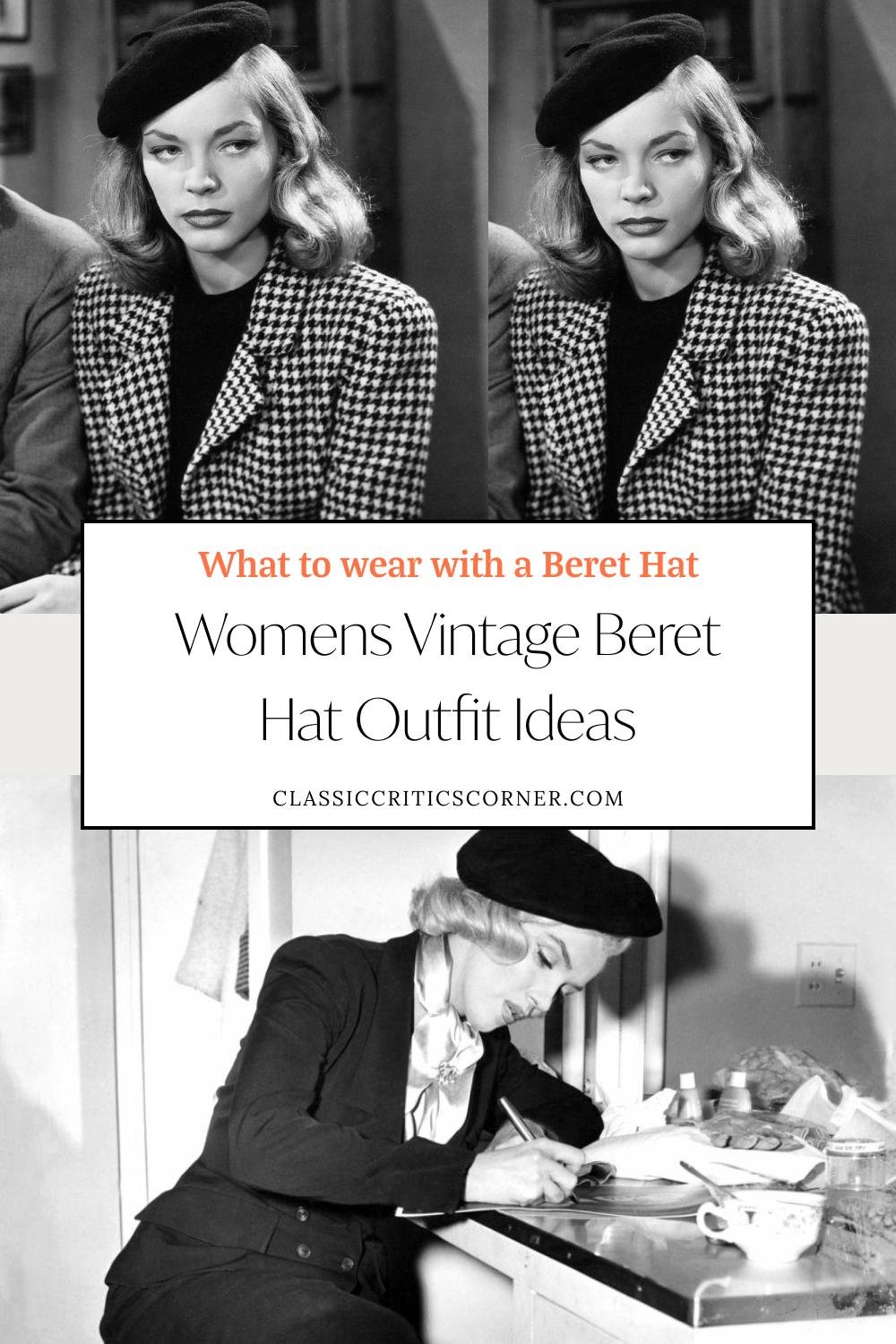The image resembles a vintage magazine ad or a book cover featuring fashion advice. At the top, there are two identical photographs of Lauren Bacall, dressed in a black beret and a black-and-white houndstooth jacket, her shoulder-length hair styled beautifully as she gazes to the side. Centered is a white text box with orange text that reads "What to Wear with a Beret Hat," followed by the title in black, "Women's Vintage Beret Hat Outfit Ideas," and the website URL, classiccriticscorner.com. Below this text box, another image from the 50s or 60s features Marilyn Monroe in a black beret and a chic black suit with a white shirt. She is depicted writing at a counter with a coffee cup nearby, creating a cohesive theme of vintage elegance.